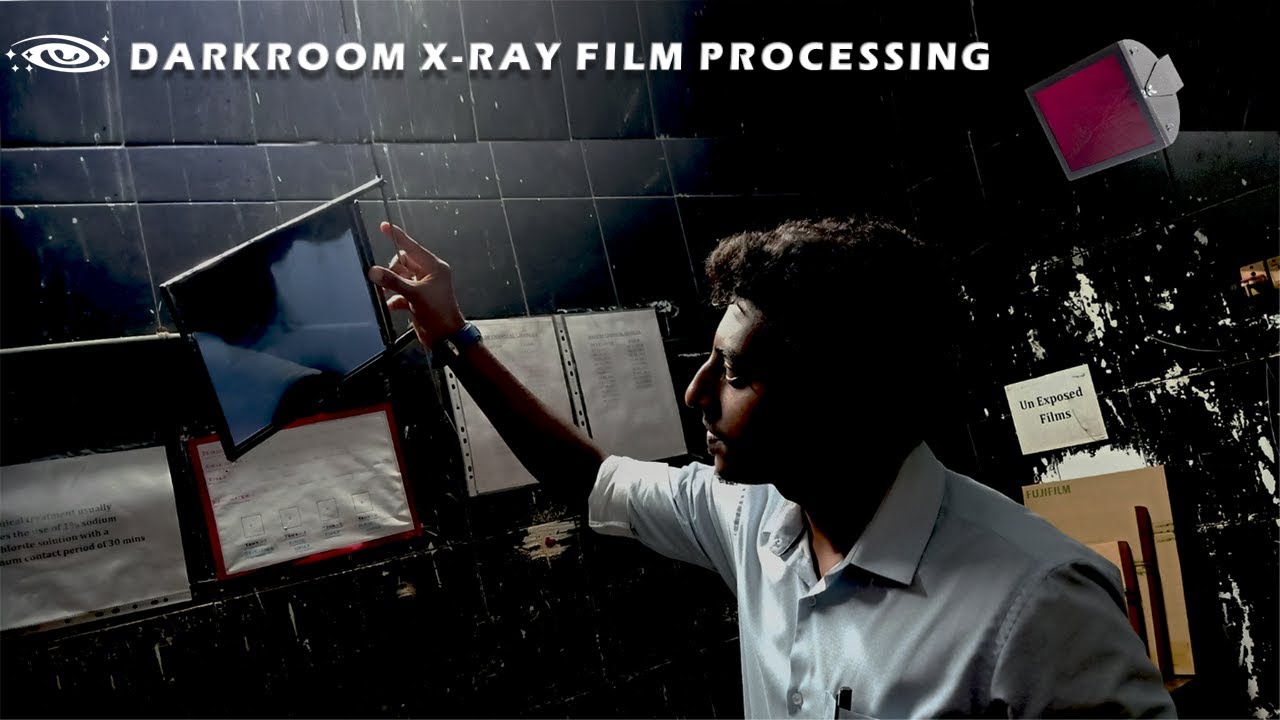In the photo titled "Dark Room X-Ray Film Processing," a dark room is depicted, complete with black tile-like walls. In the foreground, there is a man with dark skin and curly black hair, seen in profile. He is wearing a light blue, short-sleeved, button-up collared shirt. The man is holding up a translucent screen at an angle, which appears to contain a piece of x-ray film. Behind him, various sheets of film are visible, affixed to the black tiled wall. Additionally, a sign that reads "unexposed film" is noticeable. In the upper right corner of the image, a square lamp emits a reddish-magenta glow, adding to the darkroom ambiance. Various pieces of paper are also visible on the wall, suggesting educational purposes, although their exact content is indiscernible.